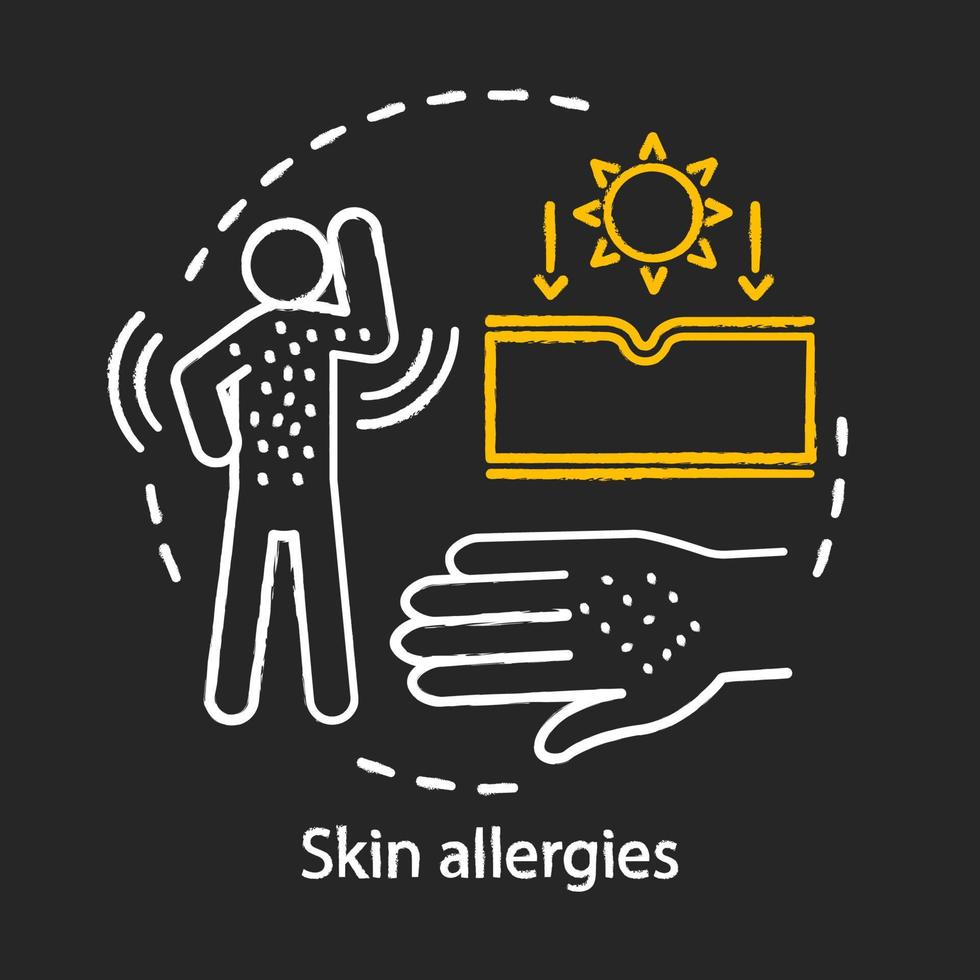The diagram, set against a black background, is an educational illustration labeled "Skin Allergies." With white and yellow marker drawings, it vividly depicts the cycle and effects of skin allergies. Starting at the top, an outstretched hand dotted with white spots illustrates an outbreak. Moving clockwise, the next element is a full-body outline of a person, displaying similar white dots on the torso and upper arms, with motion lines indicating shaking or scratching. Further clockwise is an image of the sun shining down onto a rectangular surface, representing the impact of sunlight on the skin. Completing the circle, the hand with white dots appears again, encapsulating the cyclical nature of the skin allergy process. The entire diagram is interconnected with a circular dotted line, emphasizing the recurring and pervasive impact of skin allergens.